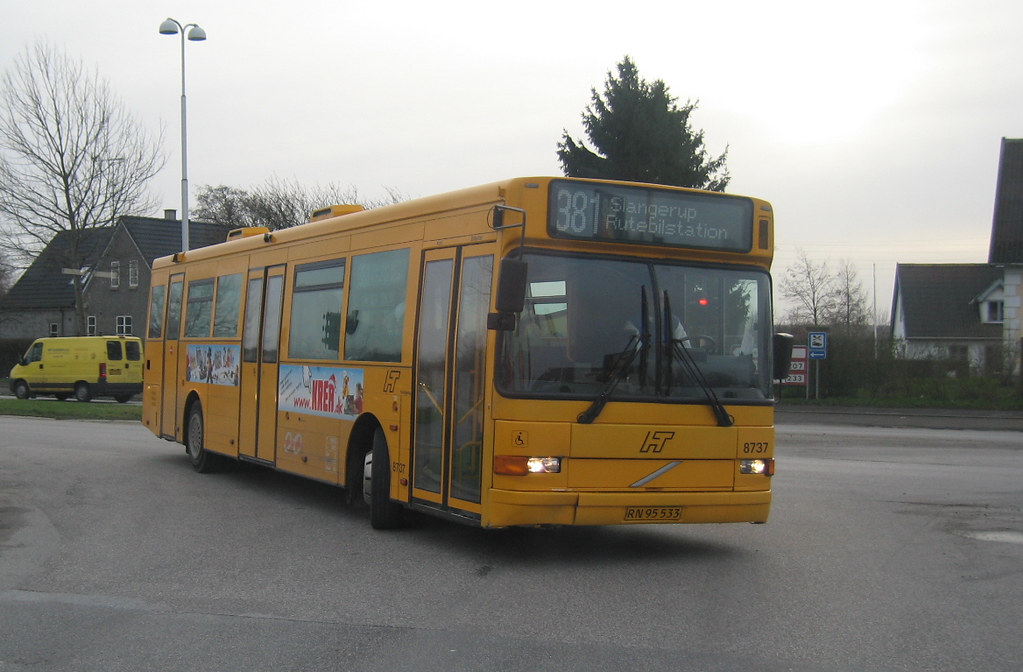This is a color photograph taken on a gray day, featuring a light orange city bus as the main focal point, which is turning towards the camera. The bus has a flat front with a digital display on top, showing "381 Slangerup Rudal Bill Station," suggesting it is likely in Europe. The bus also displays additional numbers such as "8737" above a light and has a license plate marked "RN 9553." It is equipped with three sets of doors—two double doors and one additional door in the back. On the right side, you can see several advertisements, possibly movie posters. The bus driver is visible through the front window.

In the background, there are houses: a white house with black shingles to the right of the bus and a brown house with a black triangular roof to the left. There's a yellow van trimmed in black on the opposite street, also going the opposite direction. Above the van, a white street light with dual curved lamps is visible. Additionally, there is a tree with no leaves on the left-hand side and a green-leaved tree directly behind the bus. The road the bus is turning from is light gray asphalt, and accompanying street signs can be seen to the bus's right. The sky is light gray, providing a muted backdrop to the vibrant colors of the bus and surrounding elements.